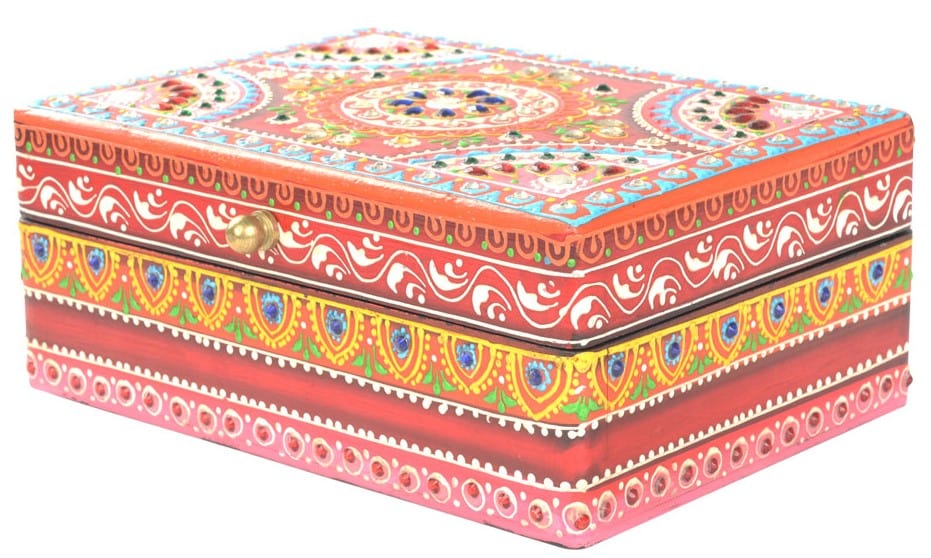The image displays a vividly colorful, intricately designed rectangular box, approximately four inches tall, six inches wide, and four inches deep. The box is adorned with multiple ornate layers, each showcasing a different pattern and color scheme. The bottom-most layer features a pink background with designs resembling berries and white dots. Above it, a narrow band presents a red and black gradient with white dots. The third layer from the bottom exhibits a vibrant combination of red, yellow, and blue segregated by dots. The box’s lid is equally detailed, starting with a red layer adorned with green dots followed by a red and white swirl pattern. At the very top, the design becomes even more elaborate with a mix of blue, red, orange, white, and green elements. A gold knob sits prominently on the main front, designed to lift the lid. Additional decorations include floral motifs and large and small circles, quarter circles with red accents, and an overall mixture of vibrant colors like red, blue, white, and pink. This stunningly decorated box, with its layers of complex patterns and rich color palette, could be mistaken for a miniature suitcase or even a non-functional, beautifully adorned mattress due to its rectangular prism shape and detailed artistry.